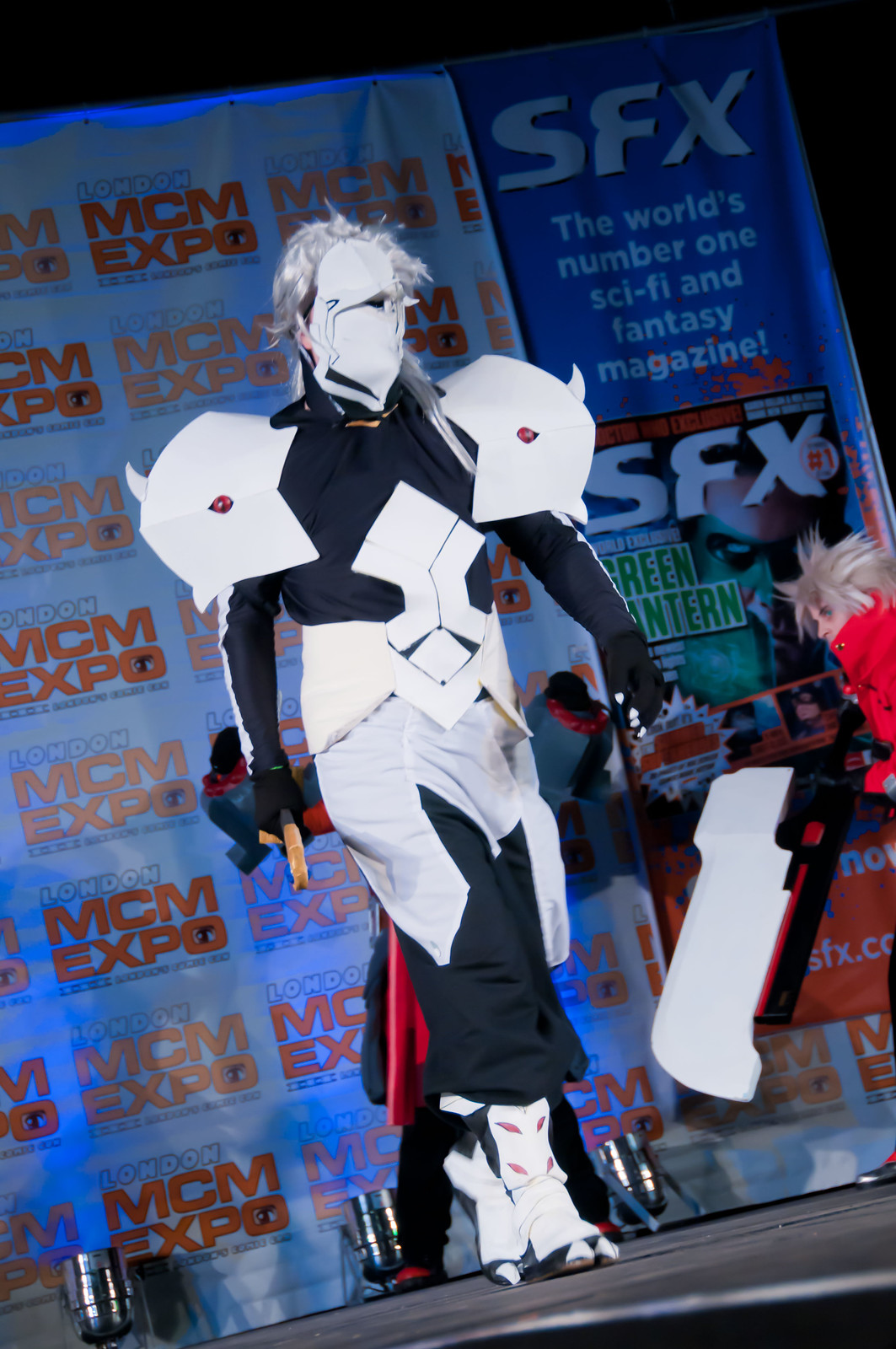This detailed portrait-mode photograph, taken at the MCM Expo in London, captures a person in an elaborate and futuristic cosplay costume, seemingly inspired by anime or video game characters, on a stage with a black surface underfoot. The backdrop is a blue banner emblazoned with "MCM Expo" and "SFX, the world's number one sci-fi and fantasy magazine."

The individual is striking a pose with their arms extended to the sides, and they are slightly tilted to the right, adding a dynamic element to the image. They are wearing a distinctive outfit featuring a gray wig and a white mask with black accents, covering most of their face except for a single central eye hole. Their costume includes massive shoulder pads resembling white helmets with red dots in the center, giving them a robotic appearance. The person's attire consists of a gray top and pants, complemented by white boots designed to mimic hooves.

Additional details include black gloves with white marks on the nails, and an intricate white design around their midsection that forms an upward-pointing arrow on their chest. A white-and-black element, possibly another character, intrudes from the right side of the image, showing a blonde-haired individual with a red scarf around their mouth, partially cut off at the neck.

In the background, another person with anime-style hair and blue contacts can be seen, adding to the lively and immersive atmosphere of the cosplay event. The detailed signage and busy stage setting help convey the excitement and creativity that permeate the event.